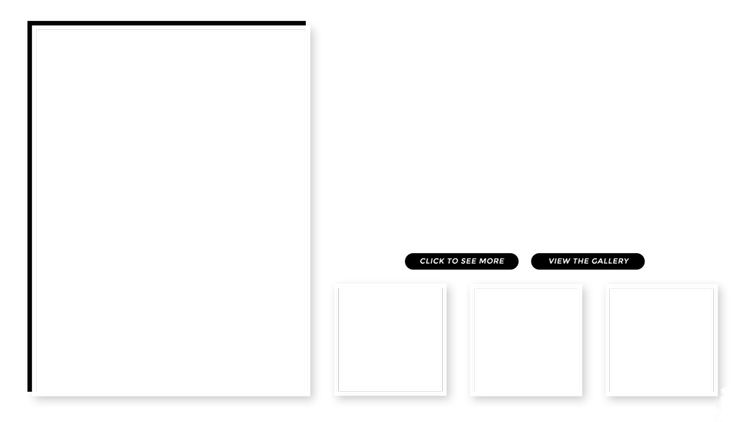The image features a total of four squares positioned against a white background, arranged in a row from left to right. The first square on the left is significantly larger than the other three and is distinguished by a black border that outlines the top and left sides, with the remaining parts shaded in light gray.

Adjacent to this large square, with a small space separating them, are three smaller squares of identical size. Each small square is designed with a white border and an inner tile-like demarcation.

Extending horizontally from the middle top edge of the first small square to the middle top edge of the second small square is a black, horizontally oriented oval. Inside this oval, the phrase "CLICK TO SEE MORE" is inscribed in capital letters with white text.

Similarly, another black oval stretches from the middle top edge of the second small square to the middle top edge of the third small square. This oval contains the text "VIEW THE GALLERY," also in capital letters and white font.

The overall arrangement creates a structured, minimalist aesthetic, with clearly marked interactive elements inviting further exploration of the content.